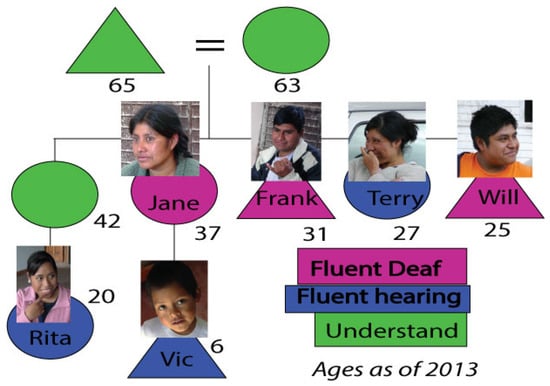The image is a detailed family tree diagram with various colored geometric shapes and portraits, representing family members and their language proficiencies. At the top, a green triangle labeled "65" is linked by an equal sign to a green circle labeled "63." This pairing gives rise to Jane, Frank, Terry, and Will in the second row. Jane, portrayed in a magenta circle, is 37 and fluent in deaf communication. Frank is shown in a magenta triangle, aged 31, and also fluent in deaf communication. Terry, in a blue circle, is 27 and fluent in hearing. Will appears in a magenta triangle, aged 25, and is fluent in deaf communication. Further connections show Jane linked to Vic, a blue triangle aged 6, indicating he is fluent in hearing. Additionally, Jane connects to Rita through a green circle labeled "42," which signifies understanding, leading to Rita in a blue circle, aged 20, and fluent in hearing. The legend at the bottom right clarifies that magenta indicates "Fluent Deaf," blue denotes "Fluent Hearing," and green signifies "Understand," with all ages referenced as of 2013. The diagram lacks any borders or background color.